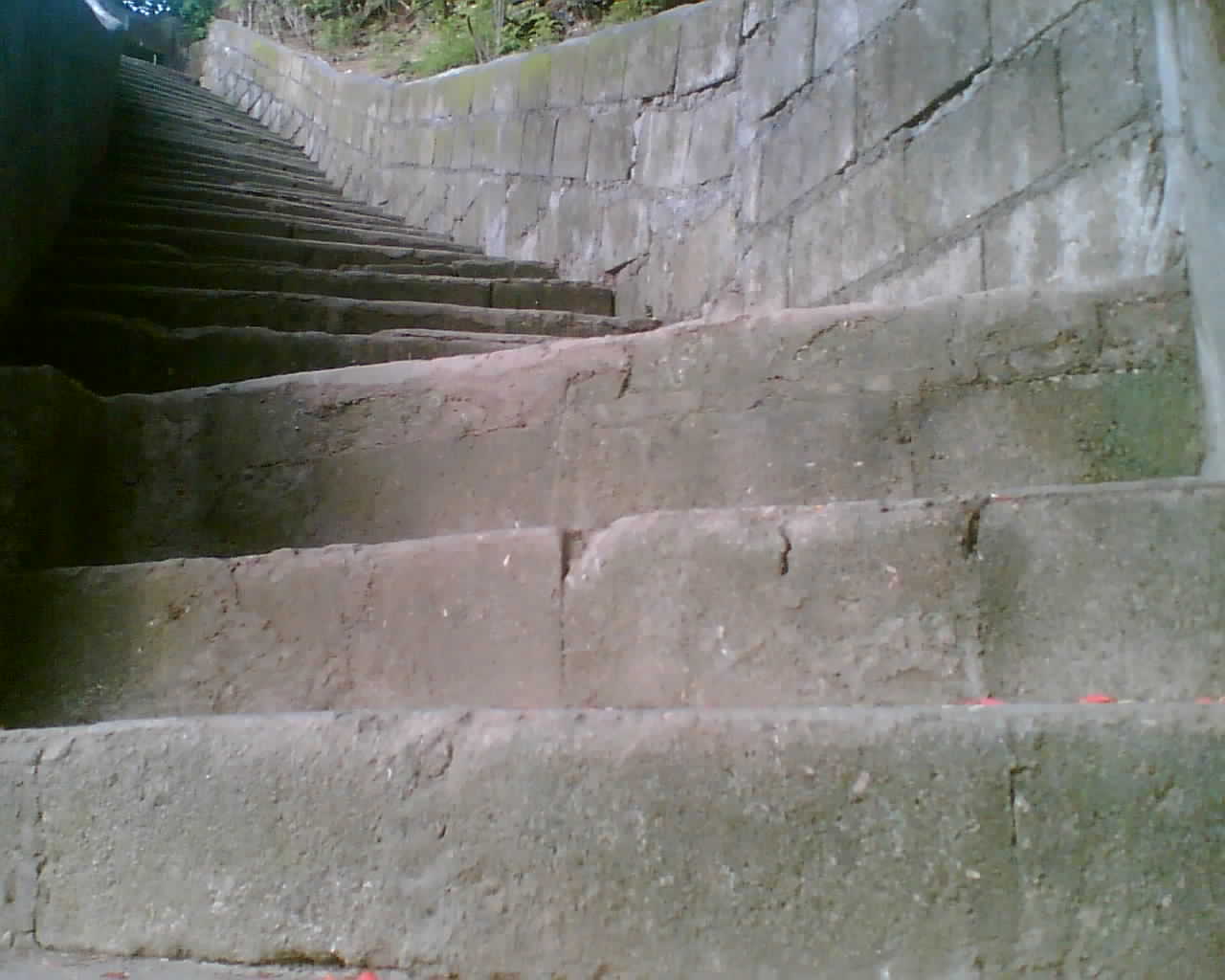This detailed color photograph, taken partially outdoors, captures an ancient, gray stone staircase ascending a hillside. Sunlight filters through, illuminating parts of the scene and casting shadows. To the right of the steps stretches a chest-high stone wall, matching the aged, weathered texture of the stairs. Green plants and shrubbery peek through in the background, adding a splash of color. The staircase consists of multiple steps, slightly angled to the upper left and seemingly continuing beyond the frame. Despite minor mold growth on the walls and earthy surroundings, the structure's historical and enduring presence is evident.